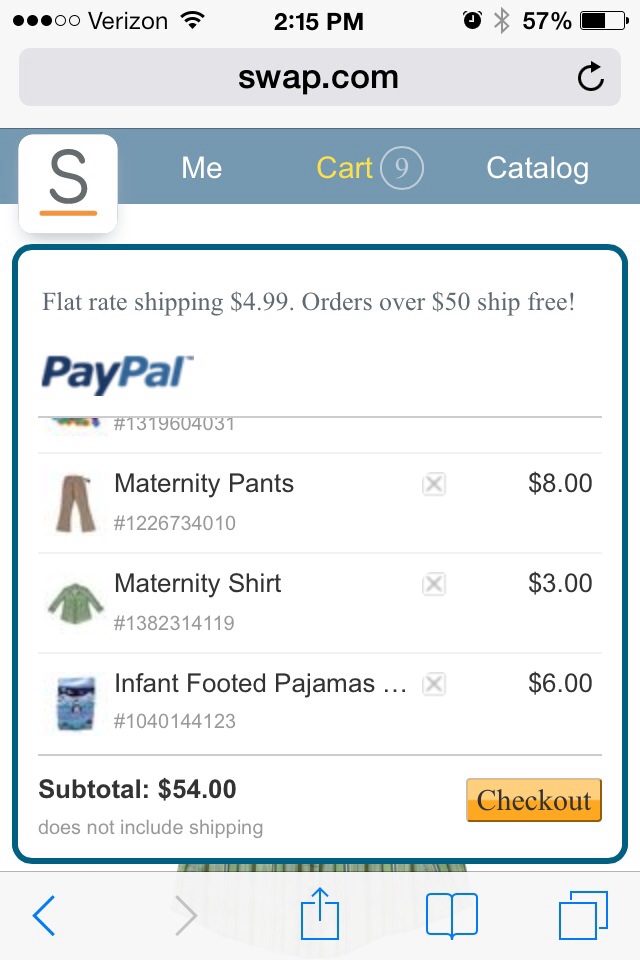The top left corner of the image displays three circles and two Holland docks. Positioned along the horizon is a clock showing the time as 2:15 PM, alongside a Bluetooth symbol and a 57% battery indicator. The webpage shown is from HedgePriceSwap.com and a refresh button is visible.

Prominently featured is an SSME cart with a yellow background. There is a highlighted item in a circular frame, associated with the number nine in the catalog, which has blue borders.

The webpage informs customers about flat-rate shipping priced at $4.99, along with an offer for free shipping on orders over $50. The text also states, “Pay a pound.”

Several numbers appear on the page, likely referencing item codes and transaction details: 1319604031, 1226734010 (return advance), and 1382314119 (an $8.00 return charge). An infant footed pajama is listed with the item code 1040144123, priced at $6.00. The shipping total is $54.00, excluding additional shipping costs.

Towards the bottom of the image, there is a yellow rectangle labeled "Checkout." The background is predominantly white. Navigation arrows (left, right, and square arrows) as well as duplicate square icons are also present, indicating potential interactive buttons or features.